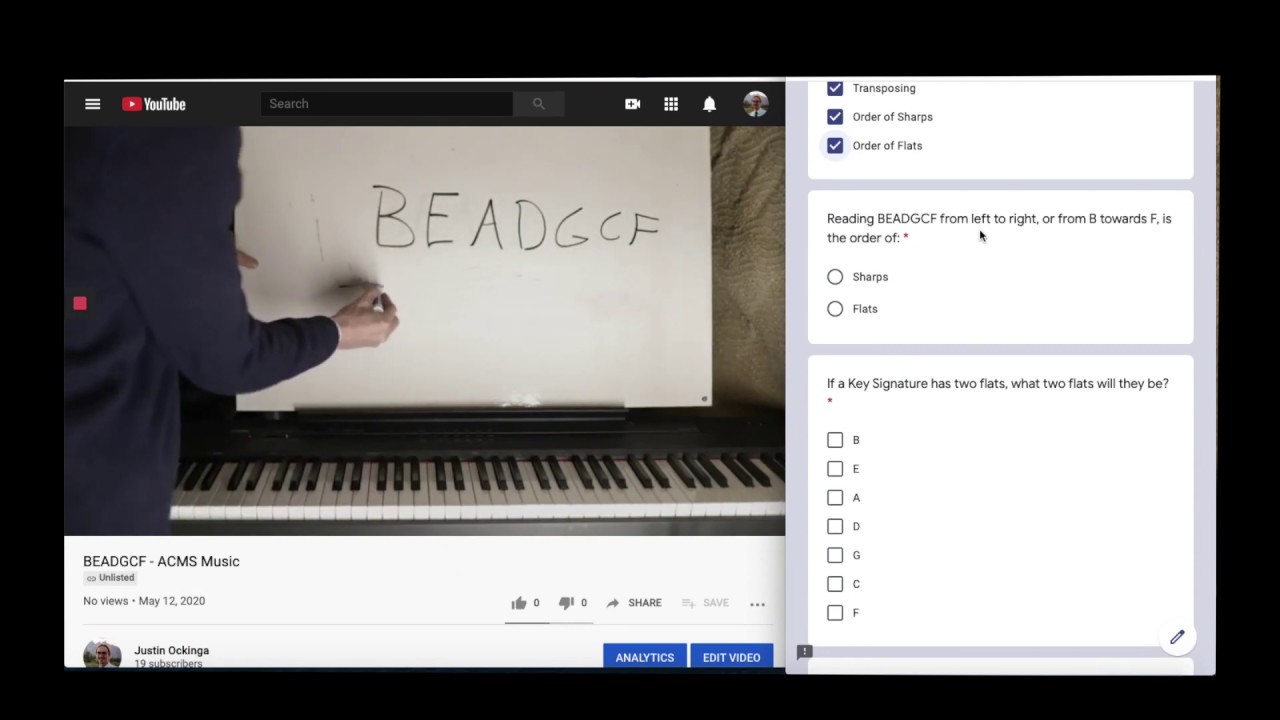A detailed caption for the described image could be:

"This image is a screenshot of a YouTube page, possibly from an educational or tutorial video on music theory. The screenshot is framed by a black border and appears small in size, necessitating zooming to read the text clearly. 

At the top left corner, there's the distinctive YouTube logo, accompanied by a search bar and some icons. The central focus of the image is a video thumbnail featuring a person wearing a blue jacket with a noticeable red spot. The individual is holding a writing instrument and appears to be drawing or writing on a piece of paper placed above a computer keyboard. On the paper, a sequence of letters 'B-E-A-D-G-C-F' is visible, potentially indicating a musical or coding sequence.

Below the thumbnail, there is text in white against a black background that reads: 'B-E-D-E-G-C-F, ACMS music.' Additional information includes 'No views' and the upload date of 'May 12th, 2020.' The video has no likes or dislikes. The uploader is identified as Judith Colunga. Beneath this information, there are buttons for 'Analytics' and 'Edit video,' highlighted in blue.

To the right of these buttons, there are several blue checkboxes related to music theory: 'Trespassing,' 'Order of sharps,' 'Order of fifths,' and 'Fifths,' followed by an instructional line: 'Read B-E-D-G-C-P from left to right or from B towards F is the order of sharps or flats.' 

Further below this section, there's a box posing a question relevant to music theory: 'If a key signature has two flats, what two flats will they be?' This is followed by a list of options, reiterating the music notation 'B-E-A-D-G-C-F.'

The content seems to revolve around music theory, specifically the order of flats and sharps in key signatures, although the precise context or the explanation within the video is not entirely clear without additional musical knowledge."